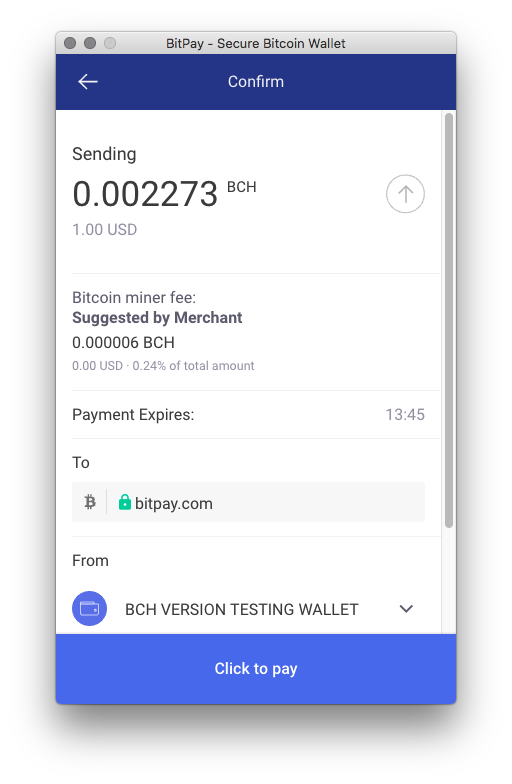This screenshot showcases the BitPay Secure Bitcoin Wallet running on a macOS interface, easily identifiable by the three iconic buttons—minimize, maximize, and close—positioned in the upper left-hand corner, differentiating it from a Windows interface where these buttons are located in the upper right-hand corner.

Dominating the top center of the screenshot is the program's name, "BitPay." Beneath the title, options to "Confirm" and an arrow to navigate back are displayed. Further down, the interface indicates an outgoing transaction, specifying the amount being sent: 0.002273 BCH (Bitcoin Cash), which is equivalent to $1 USD.

Details about the Bitcoin miner fee are provided just below the transaction amount, stating a suggested fee of 0.000006 BCH, equating to 0 USD and representing 0.24% of the total amount. Central to the page, a note indicates that the payment will expire at 13:45 (24-hour format), ensuring users are aware of the transaction's time constraints.

The bottom section includes a security indicator—a lock emblem—next to the "to bitpay.com" text, signifying that the transaction is encrypted and secure.